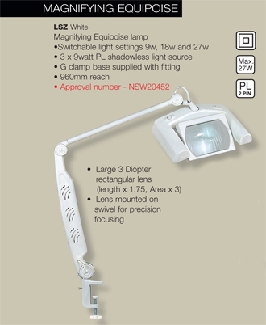In the image, a white specialized light device is displayed prominently. The light features a J-clamp at the bottom for secure mounting. The device, known as the "LSZ White Magnifying Eclipses Lamp," has its name clearly printed at the top of the image. The background is a subtle light brown, providing a neutral setting that enhances the visibility of the light.

Toward the middle section of the image, detailed specifications and features of the lamp are listed in black text, except for the approval number "NEW 20452," which is highlighted in red. The specifications include:

- Switchable light settings with options for three 9-watt configurations
- A shadowless light source
- A 960 millimeter reach enabled by the J-clamp base

At the bottom, additional technical details are provided:

- A large 3-diopter rectangular lens
- Lens dimensions of 1.5 times magnification
- A lens mounted on a swivel for precise adjustments

Next to the text, a clear picture of the LSZ White Magnifying Eclipses Lamp is displayed, showcasing its sleek design and practical features.